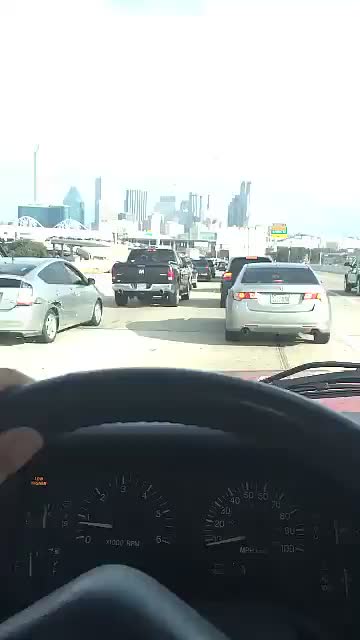The photograph captures a driver's perspective amidst heavy traffic in an American city. The bottom section of the image prominently features the black top of a steering wheel and a portion of the driver's left hand, with the thumb and part of another finger visible. In the foreground, a beige-colored street stretches ahead with several cars in view, including a silver and a black one. Beyond the traffic, a cityscape emerges into the background, showcasing towering skyscrapers against a clear blue sky. Street signs punctuate the urban scene, providing context and depth to the bustling city environment.